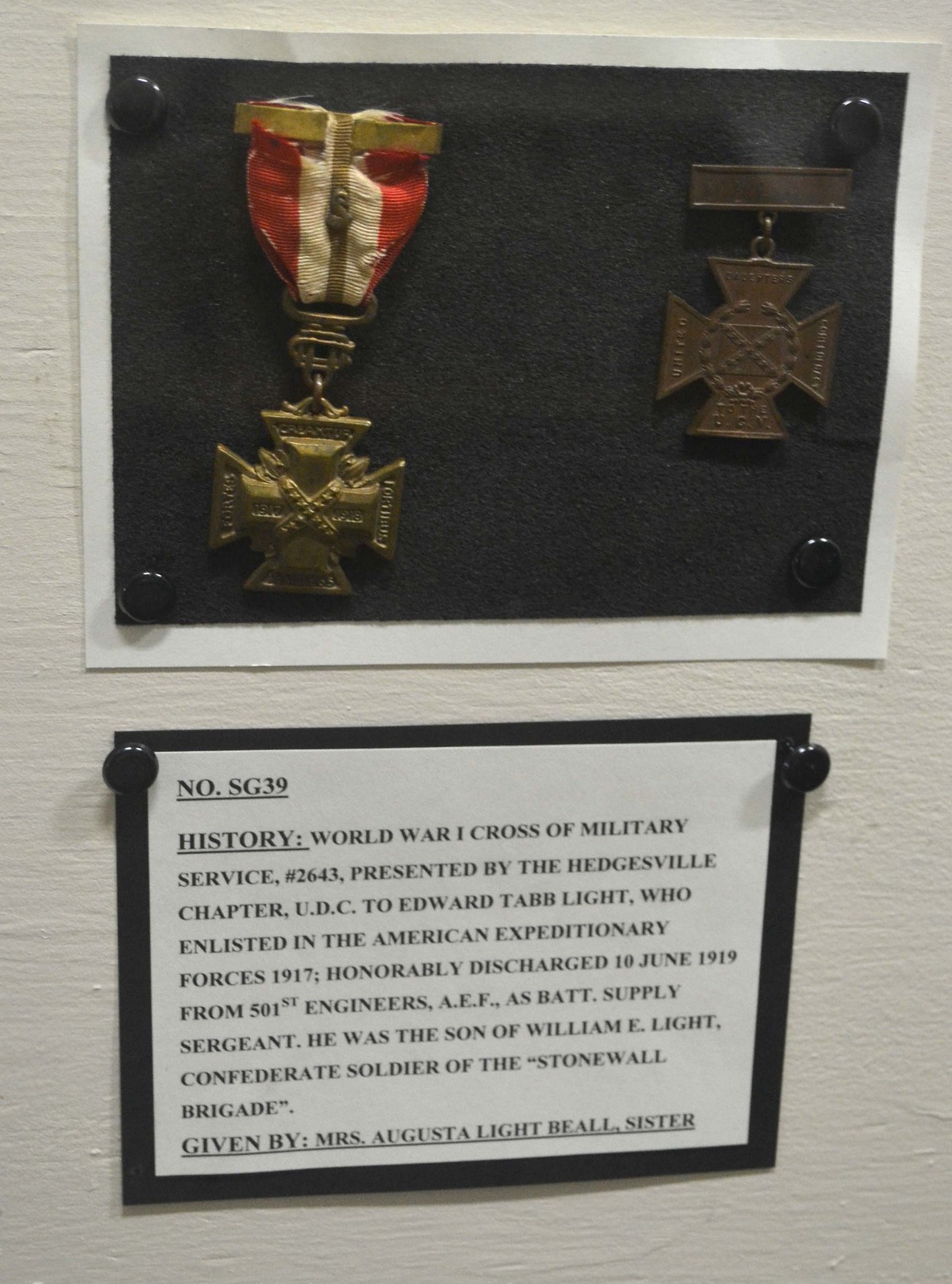This image depicts a detailed museum exhibit showcasing two World War I medals mounted on a white wall. The medals are framed and displayed one above the other, surrounded by informative text. The medal on the left has a red and white striped ribbon attached to a golden iron cross, mounted onto a black piece of fabric. The medal on the right features a simple dark bronze rectangular bar from which a bronze iron cross hangs. Below these medals, a white sign with black text provides historical context. The sign reads: "Number SG39. History: World War One. Cross of Military Service No. 2643 presented by the Hedgesville chapter U.D.C. to Edward Tablite, who enlisted in the American Expeditionary Forces in 1917 and was honorably discharged on June 10, 1919, from the 501st Engineers A.E.F. as a Battalion Supply Sergeant. He was the son of William E. Light, a Confederate soldier of the Stonewall Brigade, given by Mrs. Augusta Light Beall, sister." The medals and inscription pay tribute to Edward Tablite’s military service and familial lineage.